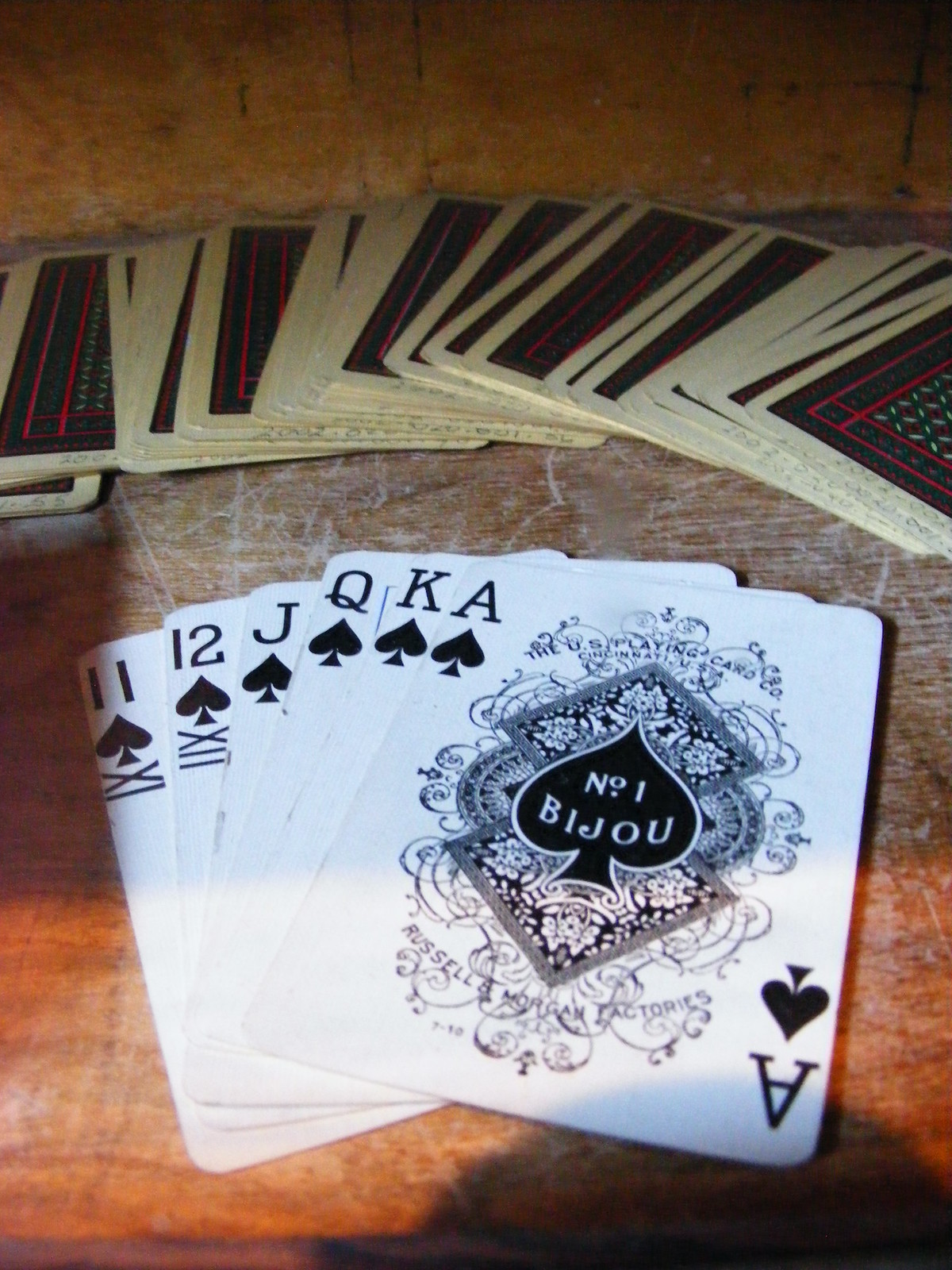This photograph captures an intricate tableau of playing cards displayed on a well-worn, scratched wooden surface. In the foreground, five cards from a Spades suit are elegantly fanned out as if held in a player’s hand. From left to right, the cards include an Ace of Spades, King of Spades, Queen of Spades, Jack of Spades, and two anomalous cards marked as the 11 and 12 of Spades. The Ace of Spades stands out with an ornate black-and-white design teeming with curly lines and geometric shapes. At the top of this design, the text reads "The U.S. Playing Card Co., Cincinnati, U.S." Above this intricate pattern rests a black spade symbol bordered in white, inscribed with "NO1 Bijou".

Directly above these fanned-out cards, a deck of playing cards is also spread out, but it reveals only the maroon and orange patterned backs of the cards. These backs are edged with white borders, which have been marked with illegible pencil scrawls, save for a few discernible numbers such as "2002-00". This striking arrangement juxtaposes the legacy of the playing cards' detailed artwork against the rustic texture of the wooden surface.